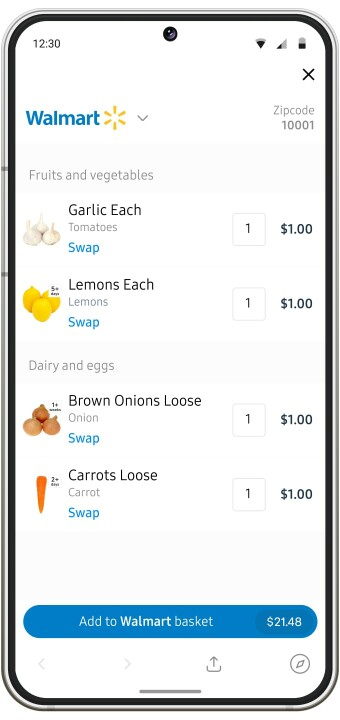The vertical image showcases the screen of a smartphone displaying a Walmart shopping webpage. Prominently visible at the top center is a small circle where the camera is located. To the left of the camera, the time is indicated as 12:30. Right below, the Walmart logo with its iconic lettering and a yellow star appears alongside the text “zip code 10001”.

Beneath this header is a categorized shopping list. The first section is titled "Fruits and Vegetables," starting with a photograph of garlic labeled "Garlic each." The text beside it shows an option to "Swap" the item, highlighted in blue, with a price listed as $1. Following this are items "Tomatoes" and another swap option in blue. Next is "Lemons each" accompanied by a picture of lemons, again featuring the text "Swap" in blue and priced at $1.

The subsequent section is labeled "Dairy and Eggs," but the items listed are "Brown onions loose" with an image of onions, followed by "Carrots loose" with an image of a carrot. Each of these entries includes the option to swap in blue text and are priced at $1 each.

The clean white background prominently highlights the content, culminating in a blue strip that runs horizontally across the bottom of the screen. This strip features the text "Add to Walmart Basket" in white, alongside the total amount of $21.48.